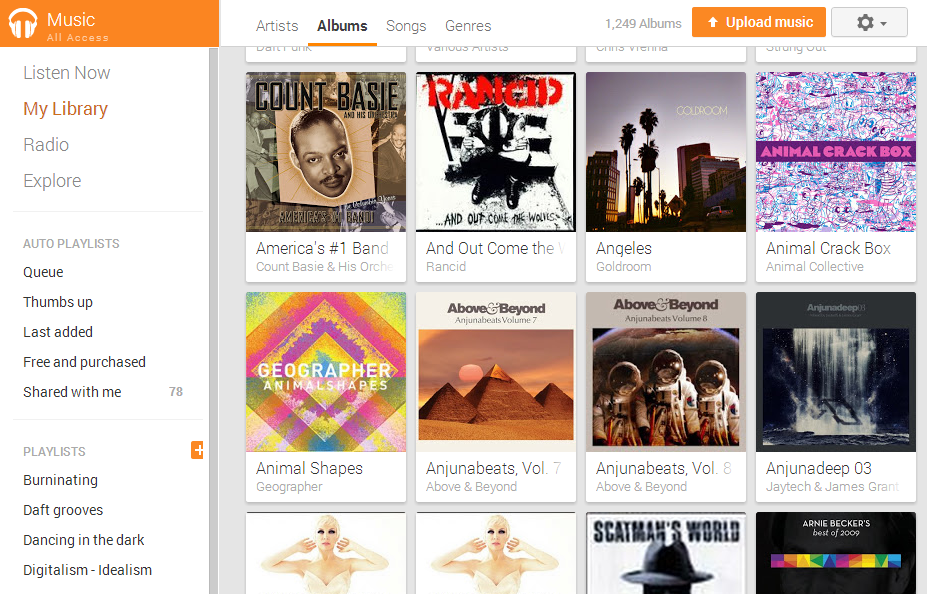Here is a cleaned-up and detailed caption for the image described:

---

Screenshot of an Amazon Music Library interface. In the top left corner, an orange banner displays "Music, All Access" beside a headphone icon. Down the left side, there is a vertical navigation column with options such as "Listen Now" and "My Library," with "My Library" currently selected. The main section on the right features rows of album cover thumbnails, four per row, with a total of twelve thumbnails visible on the screen. At the top right, an orange "Upload Music" button is present, and a cogwheel icon for settings is positioned in the far right corner. Next to the cogwheel, "1249 albums" is displayed in small gray font, indicating the number of albums in the user’s personal library. Additional categories, including "Artists," "Albums," "Songs," and "Genres," are listed on the left, with "Albums" currently selected.

---

This caption provides a thorough and clear description of the image's content and layout.